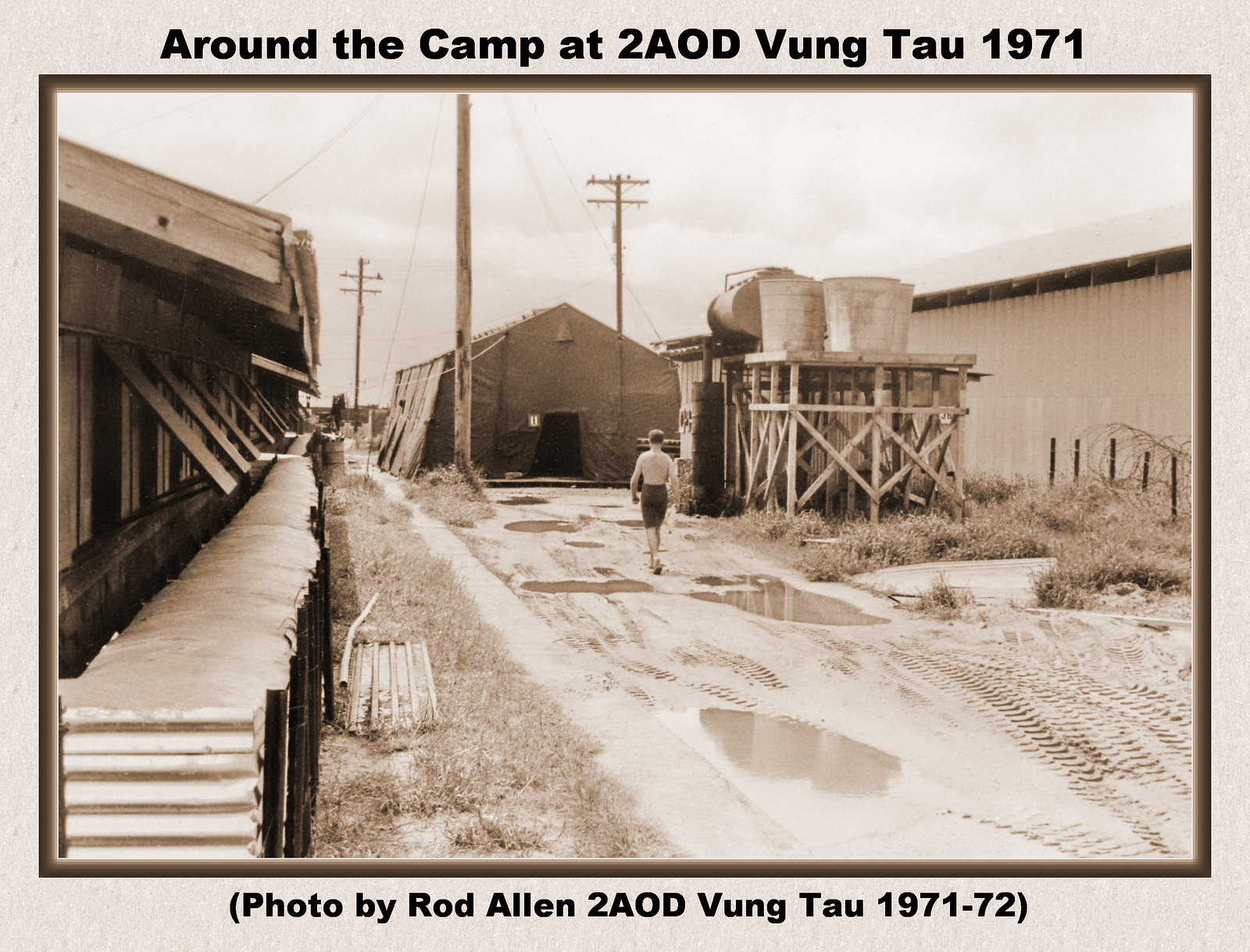This large, square sepia-toned photograph from 1971, taken at the 2AOD camp in Vung Tau, features a shirtless boy with short brown hair, wearing only brown shorts, walking away from the viewer through a muddy, puddled area. The image captures a snapshot of a likely military installation or camp, as suggested by the presence of barbed wire fences, a large tent building with an open entrance in the center, and several wooden structures to either side of him. Notably, there is a platform to his right with large buckets atop it, and a building on the far right with a barbed wire fence in front of it. The ground on the left side of the image appears to be covered in dead grass, and the sky is cloudy, contributing to the overall brown and gray tones of the scene. Additionally, the camp is marked by three telephone poles surrounding the tent and numerous tire tracks embedded in the dirt road. The bottom of the photograph is captioned with "Photo by Rod Allen, 2AOD, Vung Tau, 1971-1972," providing both a timestamp and the photographer's identity.